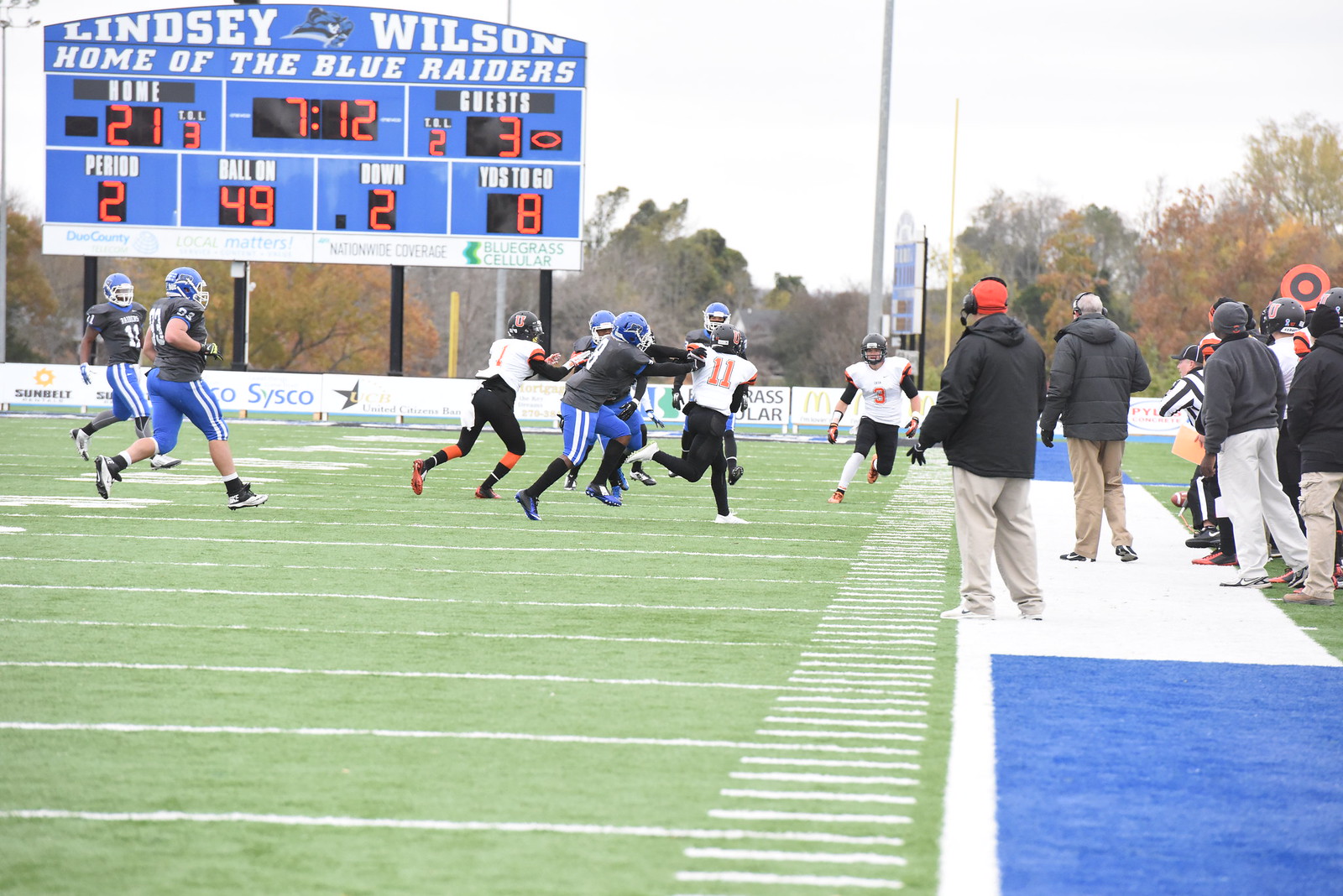This photograph captures an American football game in action, prominently featuring a dynamic play between two teams. In the center left, the team in white jerseys with black pants and black helmets appears to be on the offensive, while the defensive team is clad in dark gray jerseys, blue pants with white stripes, and blue helmets. The white-jerseyed player, likely holding the ball, is being grabbed at the center of the field by multiple players in gray jerseys. Surrounding this central tussle are approximately five players from the gray-clad team and three from the white-clad team.

The scene is set on a green football field marked with the customary painted white lines. The right edge of the image shows the sideline, painted with blue and white stripes, where coaches and assistant coaches stand, their backs turned to the camera as they focus on the game. Some members of the team in white jerseys are also visible at the edge, although mostly cropped out.

In the background, the blue scoreboard with white text reads "Lindsay Wilson, Home of the Blue Raiders," and shows the home team leading with a score of 21, while the guest team has 3. The clock displays 7:12 remaining in the second period, with the ball on the 49-yard line, second down, and 8 yards to go. The backdrop includes a tree line with autumnal colors of red, yellow, and green leaves, under an overcast gray sky.